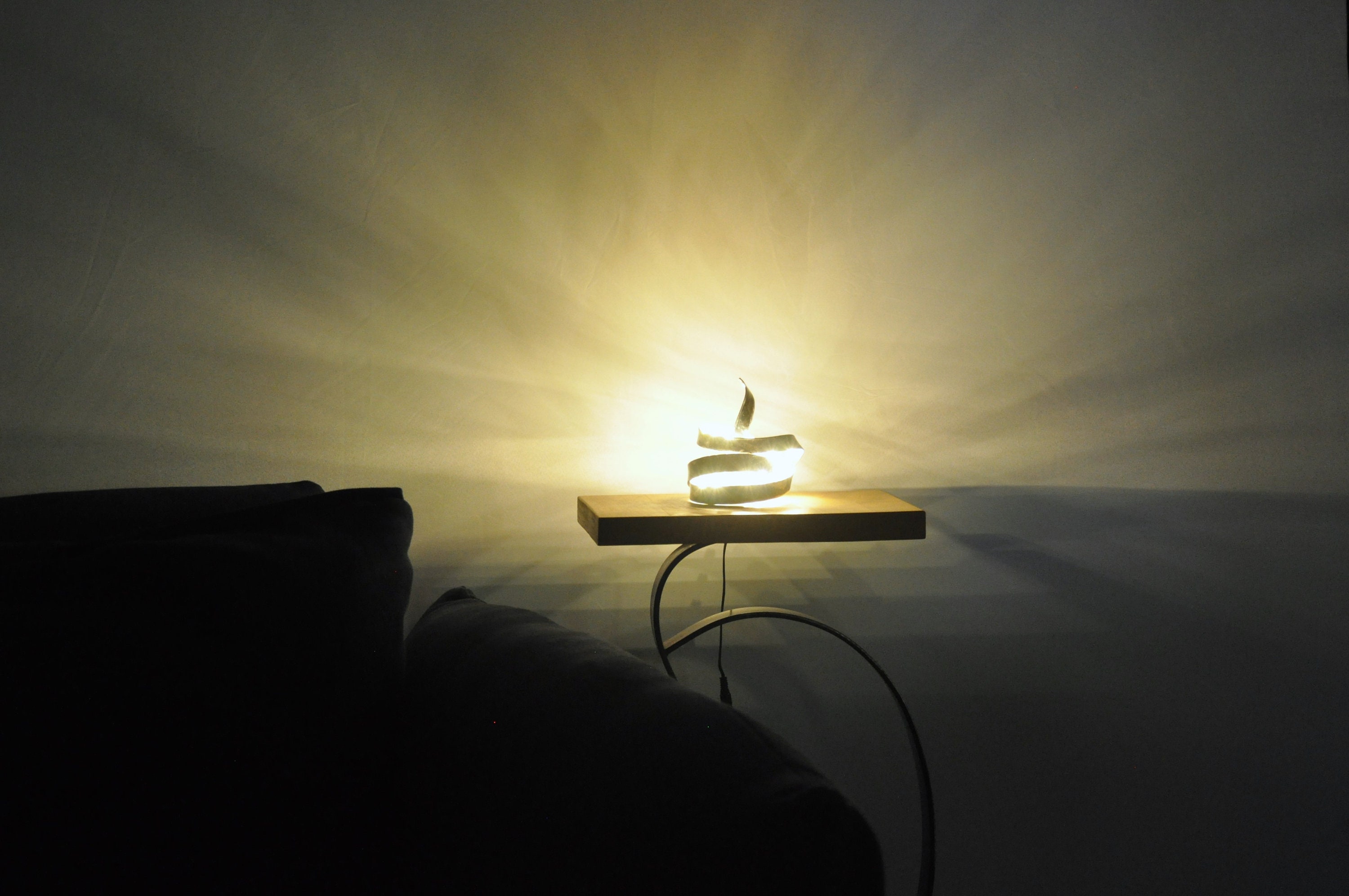This indoor photo features a cozy and intriguing corner of a room. On the left side is a dark gray, fabric couch positioned toward the viewer. Next to the couch sits a small wooden end table with a square top, supported by a curving metal leg that bends intricately beneath it. Atop the table is an ornate, spiral-shaped lamp composed of gold metal strips that radiate a warm, bright yellow light. The lamp has a cord trailing down from it and plugged into the wall, which has a bluish hue. The illumination creates a dynamic interplay of light and shadows, casting a subtle glow on the surrounding furniture and lending the entire small room a warm, shadowy ambiance.